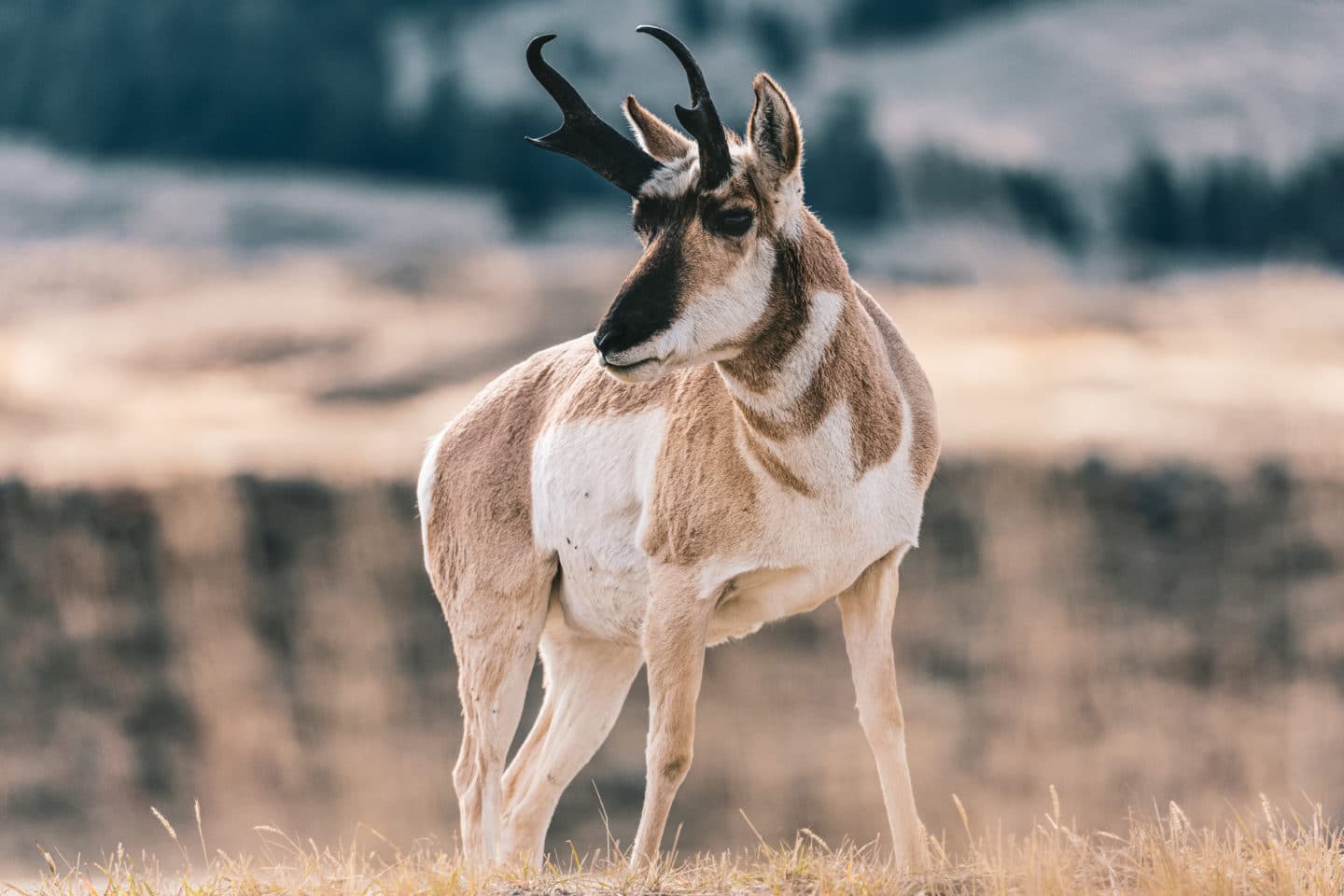In this color photograph, an animal resembling a deer or antelope stands prominently in the center of the image, captured in an outdoor environment. The animal sports two black, slightly curved horns on each side of its head, though they appear somewhat exaggerated or altered as if generated through augmented reality. It has a distinctive black nose, dark black eyes, and a white chin. The creature's face and body feature a striking pattern of light brown and white fur, with brown edging on its ears and a mix of black and white within.

The stag is posed against a backdrop that is intentionally blurred, making it difficult to discern the exact details, though hints of a black, tan, and brown landscape can be seen. The animal stands on dry, yellowish grass suggestive of a winter or savanna environment. While the scene suggests a natural habitat, the background hints at mountains and trees, contributing to the sense of an expansive field. The overall portrayal of the animal, although realistic, carries an uncanny, perhaps digitally augmented quality, particularly notable in its fur and horns.